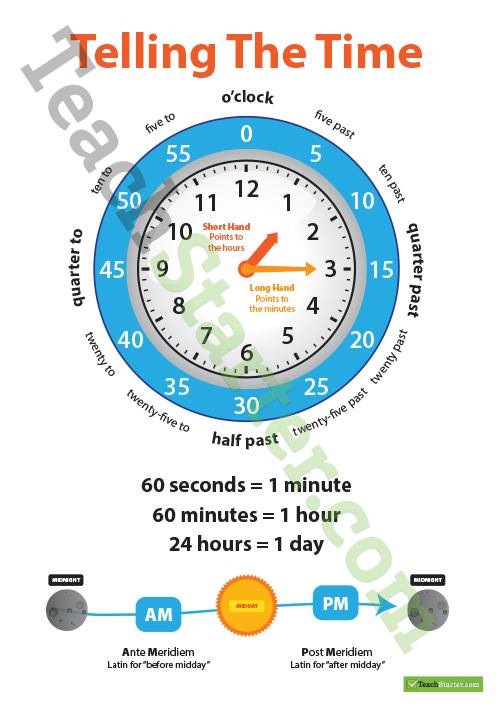The image features an educational chart designed to teach children how to read a clock. The text at the very top emphasizes the importance of practicing this skill regularly, stating, "Taking it from time to time." 

On the top left, there's a watermark belonging to TeachStarter.com. The main content of the chart is divided into various sections: 

On the right side of the chart, a neatly organized box explains the basic units of time, stating, "60 seconds equals a minute, 60 minutes equals an hour, 24 hours equals a day."

The left side of the chart provides information about the division of the day into AM and PM. The top of this section simply states "AM," defining it as "before midday," while the center section is marked as "midday." The bottom-left section identifies "PM" as "post-midday or after midday."

The central portion of the chart is labeled "o'clock" and details the positions and descriptions of various times on the clock. Starting from the top right and moving clockwise, it lists "5 past," "10 past," "quarter past," "20 past," "25 past," "half past," "25 to," "20 to," "quarter to," "10 to," and "5 to." Each of these time markers corresponds to specific positions on the clock face, going in increments of five minutes: 5, 10, 15, 20, 25, 30, 35, 40, 45, 50, and 55.

Overall, the chart is a comprehensive guide to understanding the various elements involved in reading both digital and analog clocks.